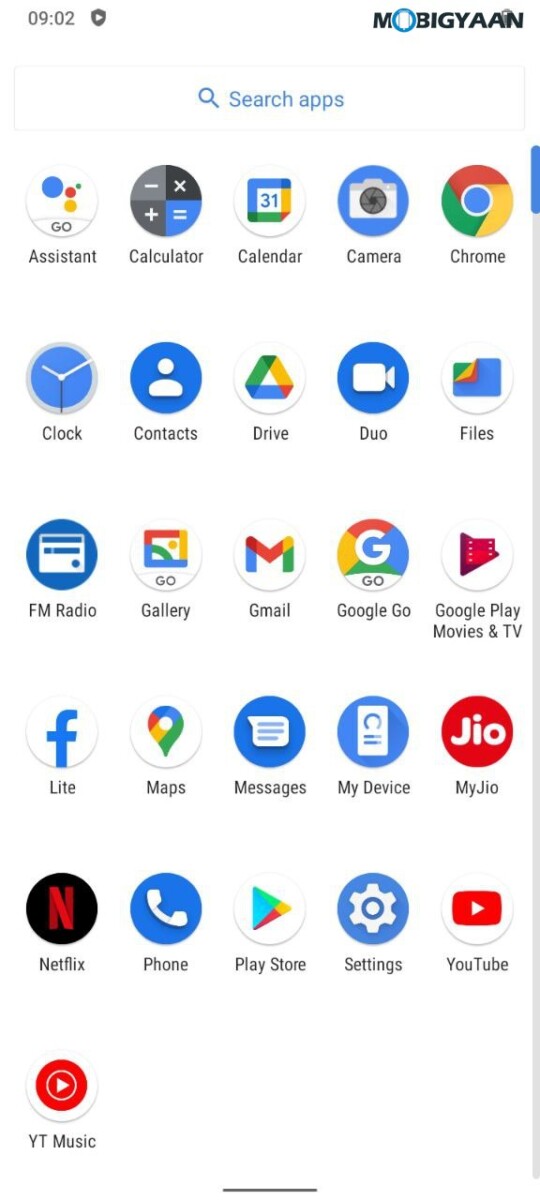This is a detailed screenshot of a smartphone's home screen. At the top of the screen, centered, is the phrase "Search Apps" in blue text. Below this, the home screen is organized into six rows of app icons, each containing up to five icons. The sixth row features a single icon. The apps displayed include, in order:
- First row: Assistant, Calculator, Calendar, Camera, Chrome.
- Second row: Clock, Contacts, Drive, Duo, Files.
- Third row: FM Radio, Gallery, Gmail, Google Go, Google Play Movies and TV.
- Fourth row: Light, Maps, Messages, My Device, My Geo.
- Fifth row: Netflix, Phone, Play Store, Settings, YouTube.
- Sixth row: YouTube Music.

The background of the screen is white. In the top right corner, the name "Moby, Guion" is displayed.